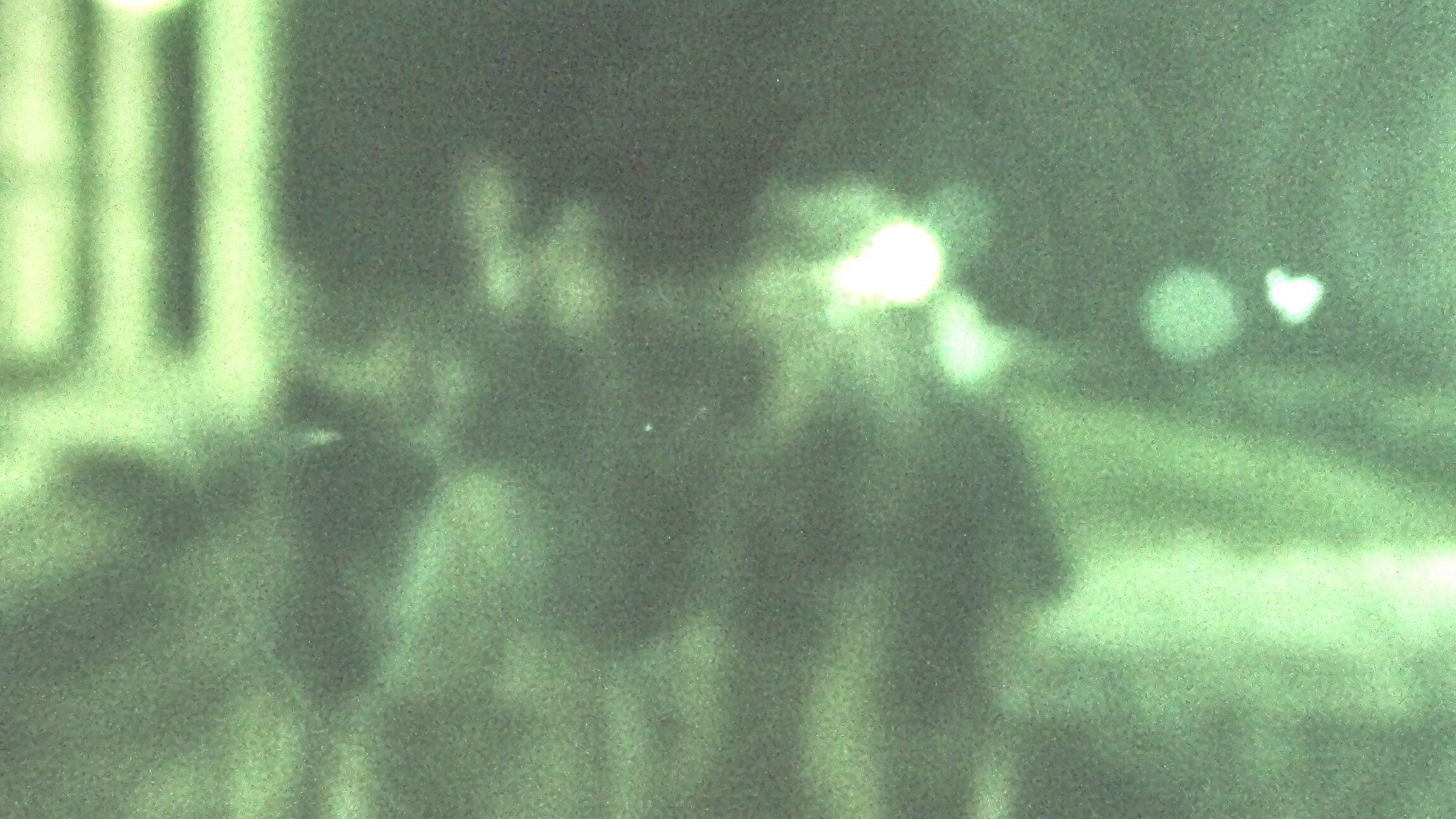The photograph is extremely blurry and dark, resembling an abstract image with indistinct details. It appears to have been taken outdoors at night, possibly through night vision goggles or a night vision filter, given the predominant green hues. The top part of the image is mostly black, contrasting with various shades of green and white light sources. In the center of the photograph, there is a bright light with a rippling halo effect around it. To the left, there appear to be some indistinct columns or perhaps the side of a building. Additionally, in the center, two faint figures can be seen. These figures, approximately the same height, could be people or animals. The figure on the left seems to have four legs, while the one on the right has an upright posture, suggesting arms and legs. Despite these possible interpretations, the image remains largely indiscernible.